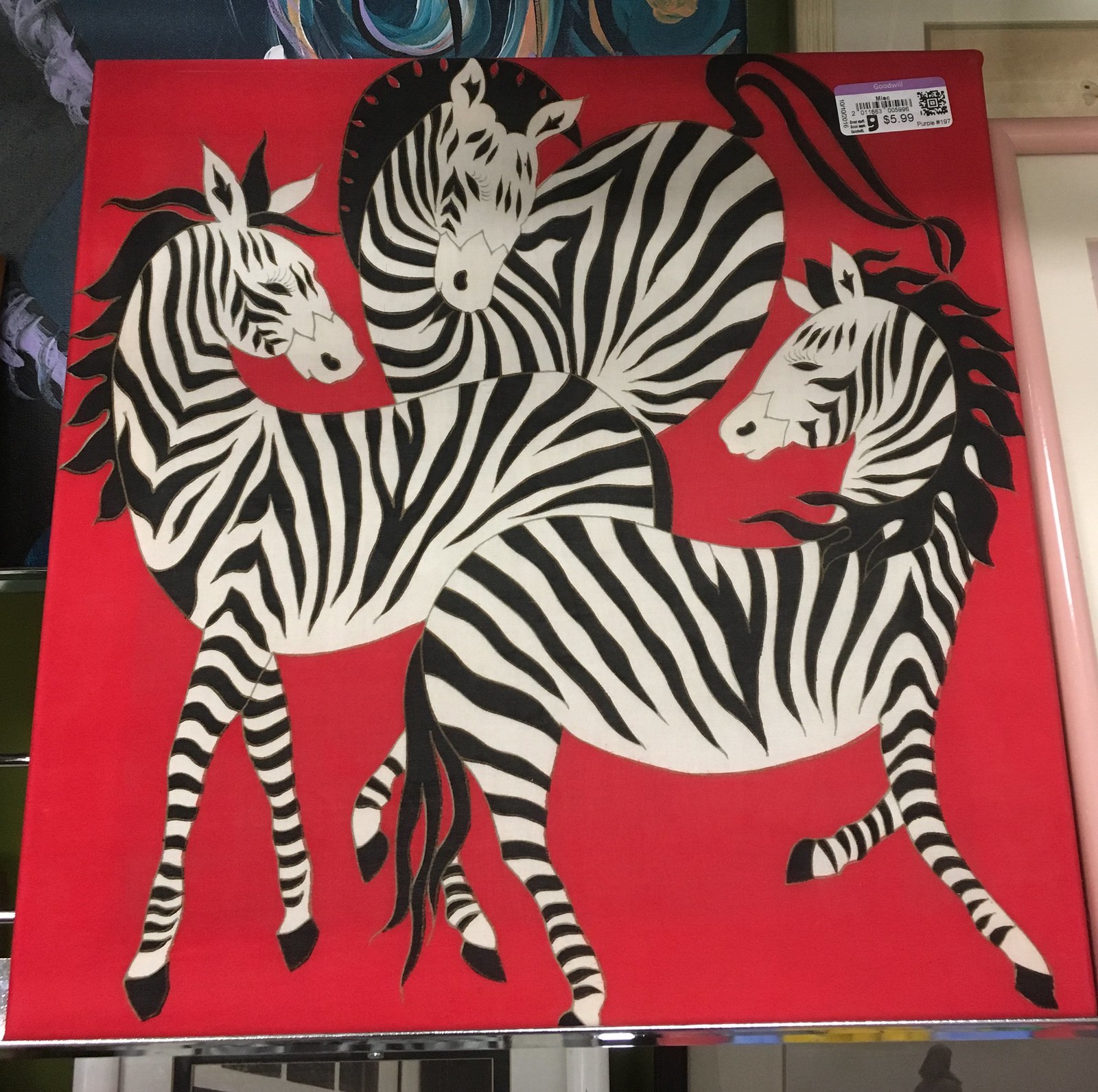This image features a large, red-painted canvas showcasing three black-and-white zebras. The zebras are arranged closely, their bodies touching in the center with their heads facing outward in different directions; one zebra's head points left, another's to the right, and the third one's is more central. Each zebra is adorned with delicate eyelashes, suggesting a feminine appearance. The canvas appears to have a chrome-like edging, potentially indicating it could be a decorative item or perhaps a framed artwork. A prominent Goodwill sticker in the top right corner shows a price of $5.99, accompanied by a QR code. In the background, partially visible, is another large portrait featuring watercolor hues of blue, purple, yellow, and orange, hinting at more artwork being displayed behind the zebra painting.